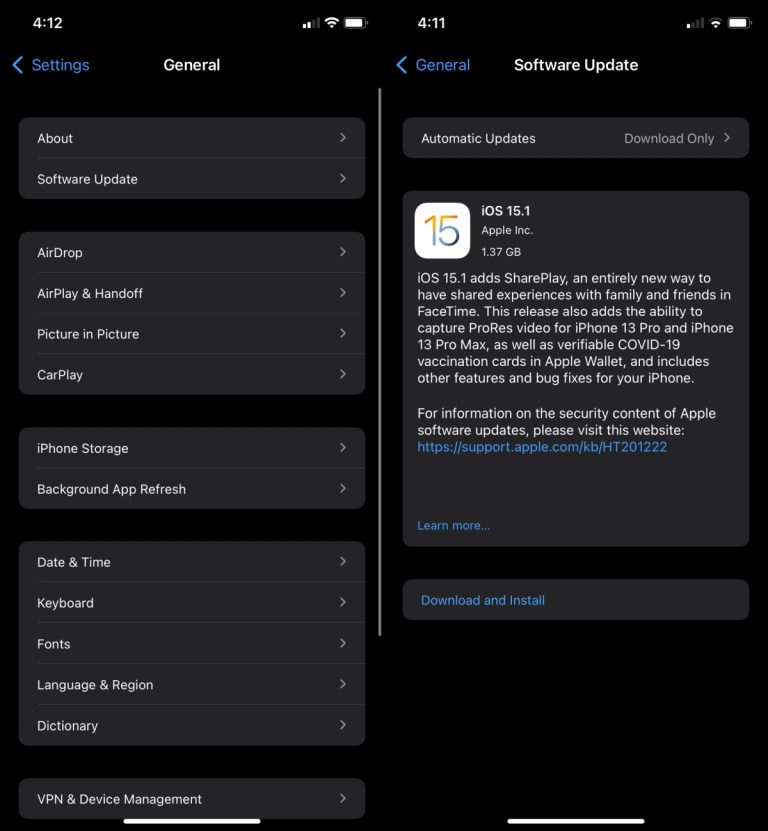This smartphone screenshot is vertically oriented, with a predominantly black background typical of device settings displays. The image is divided into two main sections, each showcasing different parts of the phone's general settings and software update functionalities.

### Section 1: General Settings Overview
- **Top Left:** Displays the time in white text, reading "4:12."
- **Top Right:** Icons indicating signal strength, Wi-Fi connectivity, and battery life.
- **Below the Time:** "Settings" is written in blue with a right-facing arrow, leading into the "General" section, displayed prominently in the center in white.

### General Settings Options
- **List of Options in Light Gray Rectangular Boxes:**
  - About
  - Software Update
  - AirDrop
  - AirPlay & Handoff
  - Picture-in-Picture
  - CarPlay
  - iPhone Storage
  - Background App Refresh
  - Date & Time
  - Keyboard
  - Fonts
  - Language & Region
  - Dictionary
  - VPN & Device Management

Each option is accompanied by an arrow, denoting the ability to click for more detailed information.

### Section 2: Software Update Details
- **Time:** Now reads "4:11" in white at the top left, suggesting information was updated slightly differently or taken at a different moment.
- **Icons:** Shows updated signal strength, Wi-Fi, and battery life indicators at the top right.
- **Main Heading:** "General" is displayed, with "Software Update" directly below it in white.
  
#### Detailed Software Update Information
- **Automatic Updates:** Displayed in a light gray, rounded rectangular box with the text "Download Only."
- **iOS Version:** Details iOS 15.1 by Apple Inc., with a size of 1.37 GB.
- **Further Information:** Description text provides information about iOS 15.1, displayed in white.
- **Web Address:** A clickable blue link for "Learn More," followed by options for "Download and Install."

The screenshot effectively communicates the current settings and update options available on the device, with a clear, structured layout for ease of navigation.